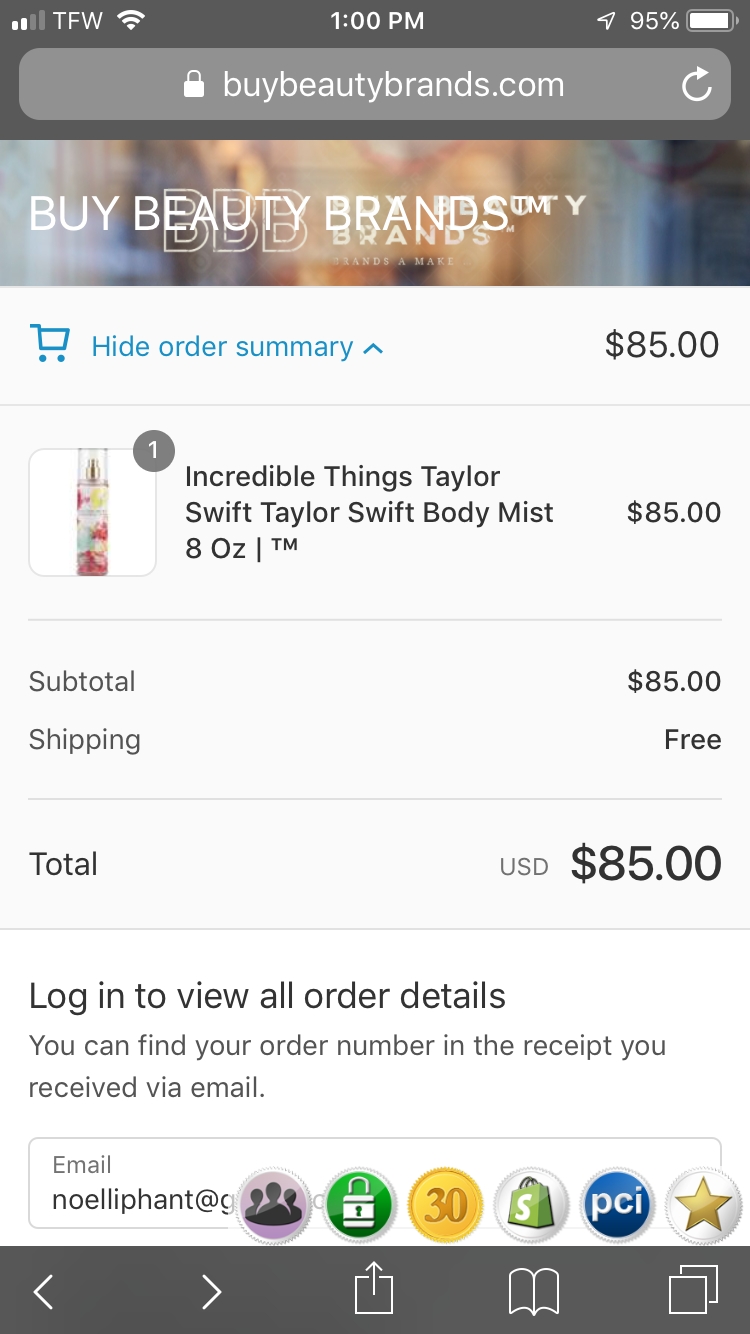The image showcases a mobile app screen displaying an order summary. The top of the screen features a gray status bar that includes an indicator showing a 2 out of 4 cellular signal strength with the label "TFW" in white, a full Wi-Fi signal icon, and a battery icon indicating 95% battery life, followed by the time displayed as "1 p.m."

Directly beneath the status bar, a banner in a mix of blue and orange hues features the white text "Buy Beauty Brands™," with the website address "BuyBeautyBrands.com" positioned above it. Below this, there is an option labeled "Hide Order Summary," accompanied by a shopping cart icon and a total amount of $85.

The main section of the order summary displays an image of a fragrance spray or body mist. The product details read: "Incredible Things Taylor Swift Body Spray," priced at $85 for an 8-ounce bottle. The subtotal is listed as $85, with free shipping, making the total also $85. The screen prompts the user to "Log in to view all your orders," and provides instructions to find the order number in the receipt received via email addressed to NOELLIPHANT, obscured partially by icons representing a lock, a coin, a shopping bag, and a star.